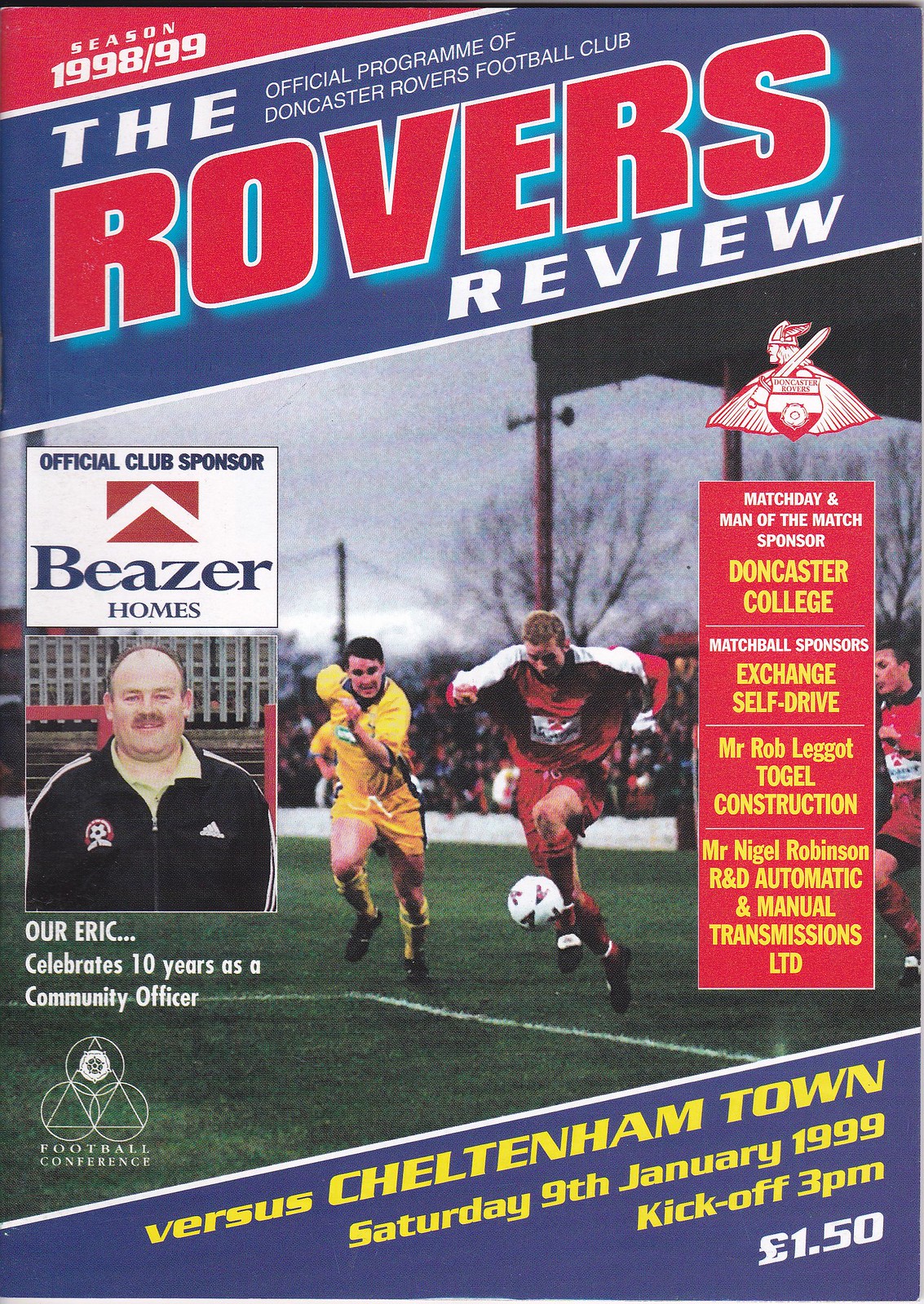The cover of the football program "The Rovers Review" for the Doncaster Rovers Football Club, features a vivid photograph of a soccer field with two men in action. One player, dressed in a red and white uniform, is in the process of kicking a white soccer ball while a player in a yellow uniform runs beside him. The backdrop includes a green field, emphasizing the dynamic motion. The top of the cover is adorned with a red, white, and blue header that proclaims "Season 1998-99," and the title "The Rovers Review" is displayed prominently in bold red letters with a blue diagonal banner. The right-hand side provides information about the match and the sponsors, while the left-hand side highlights the club's official sponsor, Beezer Homes, accompanied by a photograph of a man named Eric, celebrating his 10 years as a community officer. At the very bottom, in striking yellow print, it details the match against Cheltenham Town on Saturday, January 9th, 1999, with a kickoff time of 3 p.m. and an entry price of £1.50.